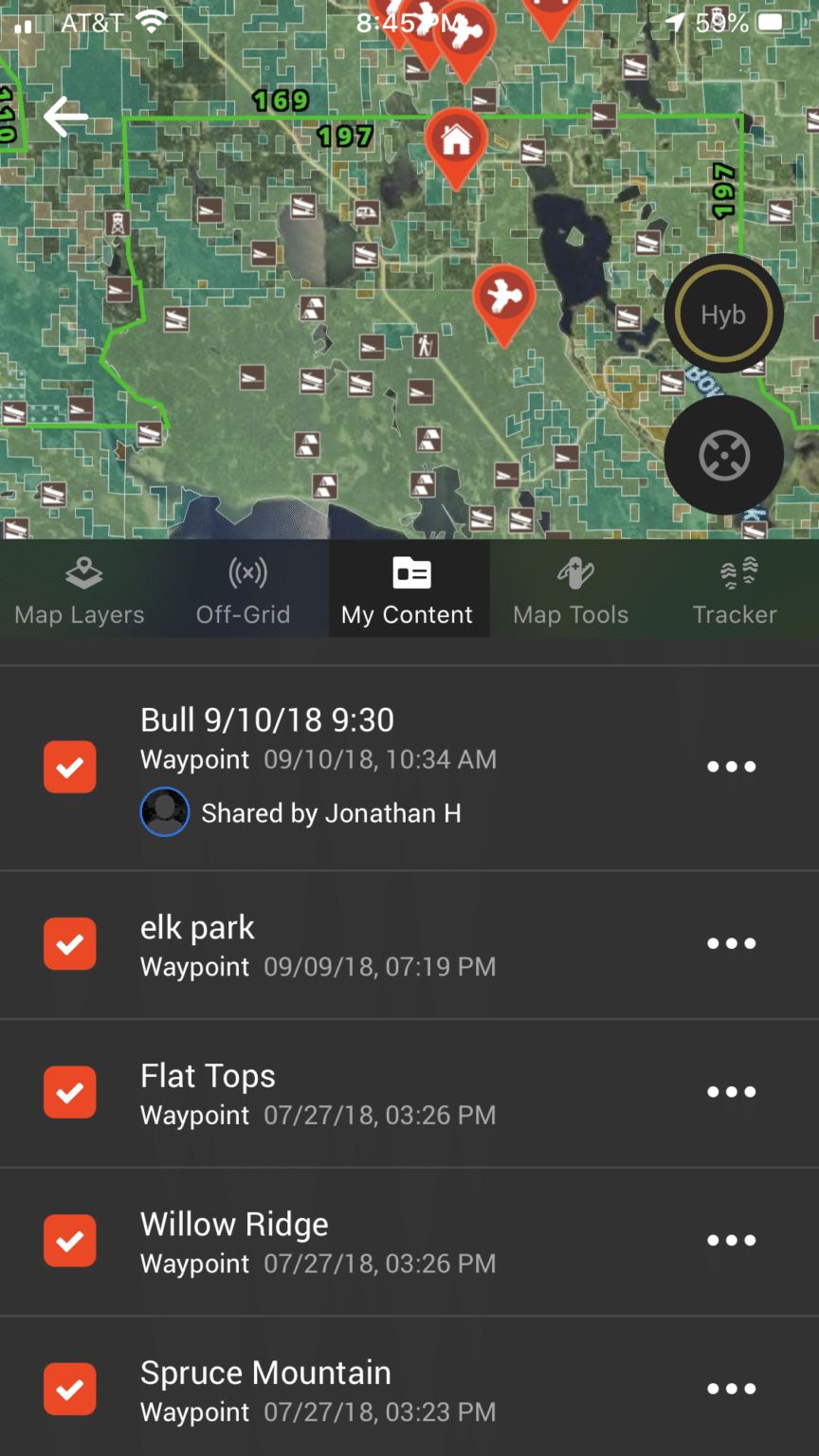Screenshot of a map interface showing multiple location symbols and waypoints. There are two highlighted circles labeled "HYB" and an unspecified location icon. At the top of the screen, the status bar displays the time (8:57 PM), battery life (59%), and the carrier (AT&T). A white arrow pointing to the left is visible, possibly indicating a navigation option. The map layers are turned off, and the "My Content" option is selected, displayed with a prominent black square background amongst gray ones. Additional features displayed include Map Tools and Tracker. The interface shows a date and time stamp format (e.g., "9/10/18 10:34 AM") for shared waypoints, mentioning specific details such as:

- "Waypoint 9/10/18 10:34 AM shared by Jonathan H",
- "Elk Park Waypoint 9/9/18 7:19 PM",
- "Flat Tops Waypoint 7/27/18 3:26 PM",
- "Willow Ridge Waypoint 7/27/18 3:26 PM."

The map interface presents a tool-rich environment designed for location tracking and navigation, with various user-generated waypoints marked and shared over time.